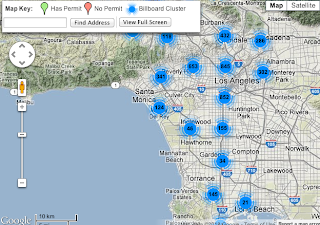The image depicts a web page showing a detailed map focused on Los Angeles and its surrounding cities. In the top left-hand corner, there is a map key indicating that green represents areas with permits, red denotes areas without permits, and blue signifies billboard clusters. Below the map key, there is a search bar that allows users to type an address and either press "Find Address" or view the map in full screen. 

In the top right-hand corner, users have the option to switch between map view and satellite view. The map prominently displays the Los Angeles area, which is heavily marked with blue clusters indicating billboards. Specific counts of billboards are highlighted, such as Long Beach with 21, Glendale with 432, and Monterey Park with around 300 billboards. However, there are no visible indications of permits within this particular screenshot, even though the key suggests that such information is available.

Users can navigate the map by panning right, left, up, or down. This detailed screenshot, provided courtesy of Google, allows for an in-depth exploration of billboard distributions across the Los Angeles area.